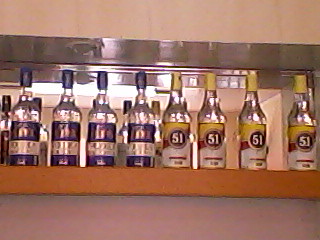This color photograph captures a detailed view of a wooden shelf adorned with a collection of eight clear glass liquor bottles, meticulously arranged in two distinct groups. The shelf is situated against a wall that transitions from a beige hue at the top to a greyish tone at the bottom due to varied lighting. A metal indent with a line runs across the entire shelf, adding a reflective, silver element.

The four bottles on the left are distinguished by large bluish stripes, blue corks, and a blue base. A long fluorescent light behind these blue bottles casts a luminous glow, enhancing their appearance. The four bottles on the right showcase vibrant yellow emblems with a prominent '51' on their labels, accompanied by maroon and white accents, and topped with yellow corks. Each of these bottles features lettering within bluish circles outlined in red, with additional small red writings on a white background.

The scene has a mirrored backdrop, likely simulating a bar or restaurant setting, reflecting both the bottles and the wall above the shelf, creating an illusion of depth and repetition. The seamless alignment and clarity of the bottles against the intricate display contribute to the captivating composition of the photograph.